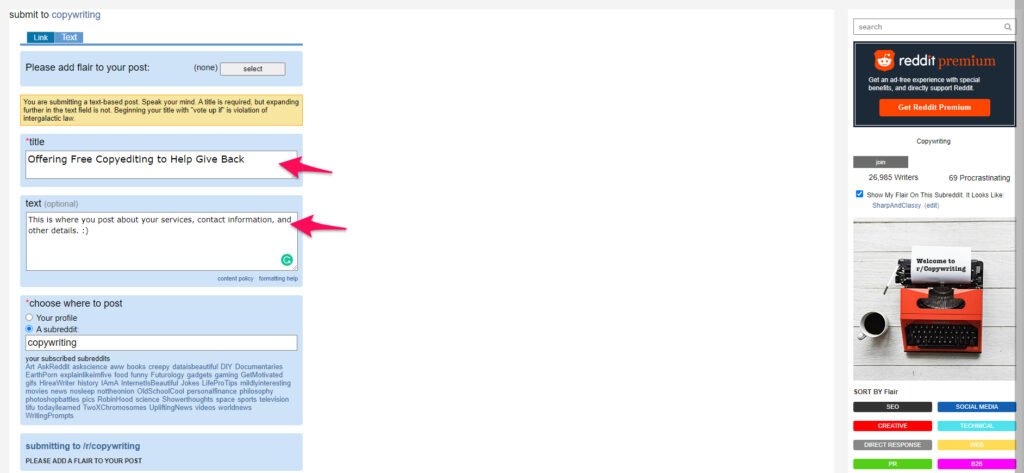The image displays a user interface for submitting a copywriting post. In the upper-left corner, a header reads "Submit to Copywriting." Directly beneath it, two fields are marked by red arrows, seemingly added using photo editing software. Between these arrows, a prompt states, "Please add flair to your post," followed by "None" in parentheses and a "Select" button. Below this section, another message reads, "You are submitting a text-based post. Speak your mind," indicating that while minimal text is required, users are encouraged to elaborate further in the provided text field.

An advisory note emphasizes that beginning the title with "vote up" violates intergalactic law. The title of the post, "Offering Free Copy Editing to Help Give Back," is visible. Further down, an optional text area invites users to share details about their services, contact information, and other relevant details. Both of these fields are targeted by the red arrows.

At the bottom, the user is prompted to choose where to post. Options include posting to their profile or a subreddit. The "subreddit" option is highlighted with a blue circle, filled in, and the specific subreddit indicated in the data field is "copywriting." A list of subscribed subreddits is also displayed for user selection.